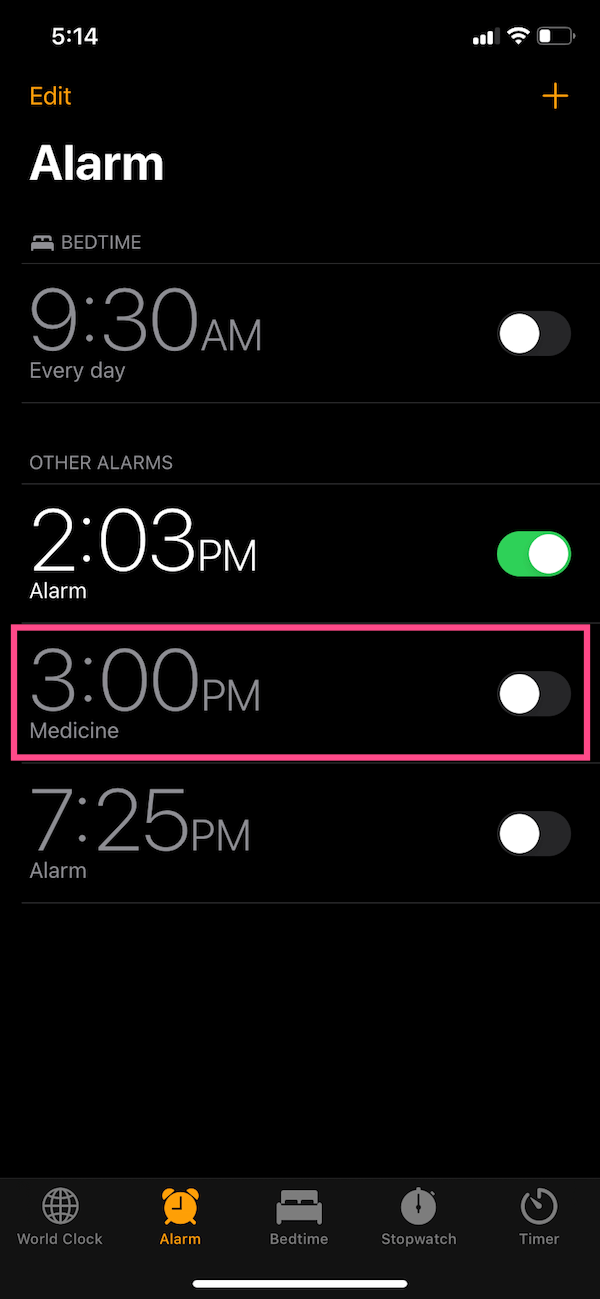In the image of the smartphone screen displaying an alarm application, the background is a sleek black. At the top left, an orange "Edit" button is prominently visible, while a "+' add button is situated on the top right. The main page text of the alarm app is predominantly white, with some grey text indicating inactive elements.

Just below the "Edit" button, the app lists different sections and scheduled alarms. Starting from the top, it displays "Alarm" and "Bedtime", followed by an alarm set for 9:30 AM that is greyed out, indicating it is off and set to repeat every day.

The next alarm listed is for 2:03 PM, which is active. This is confirmed by the green circle switch pushed to the right. Below that, another alarm is set for 3:00 PM labeled "Medicine". It is turned off, denoted by the grey colour and is outlined in pink. The final alarm listed is set for 7:25 PM and is also off.

At the bottom of the screen, there are several navigation tabs: "Clock" on the far left, followed by "Alarm", "Bedtime", "Stopwatch", and "Timer" on the far right. While these buttons are generally grey, indicating inactivity, the "Alarm" button is highlighted in orange, showing it is the currently selected tab.